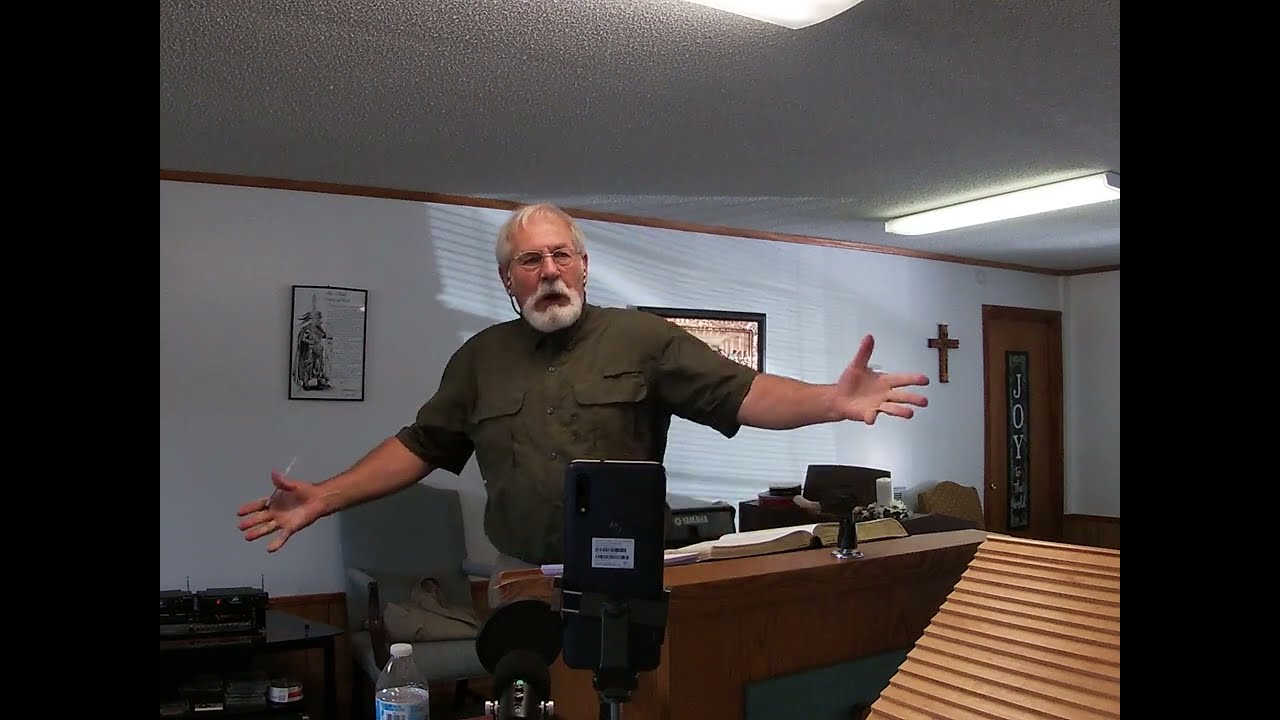In the image, an older white man with white hair, a goatee, and glasses is captured mid-sentence with his arms outstretched in a gesture that suggests he is either emphasizing a point or expressing frustration. He wears a short-sleeved, military green shirt and stands behind a lectern-like object with a bottle of water nearby. The setting appears to be religious, as indicated by the cross on the wall and the word "Joy" spelled out in white letters on a door with a glass window. Additionally, a desk with an open book, likely a Bible, and a computer monitor can be seen in the background. There is also a framed picture of the Last Supper on the wall, further reinforcing the religious atmosphere.